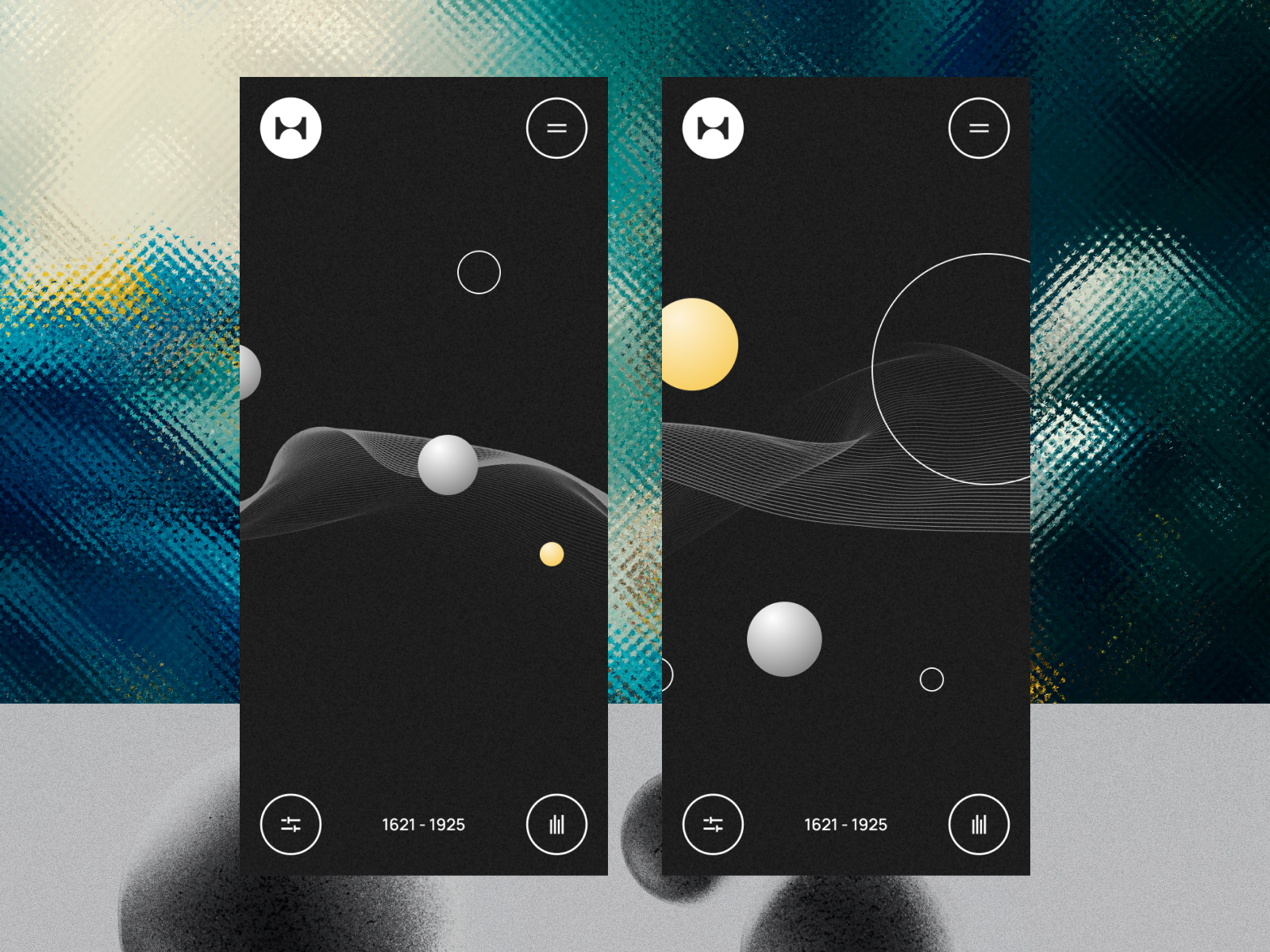This is a detailed photograph taken indoors, capturing two abstract art panels, possibly in a studio or museum setting. The backdrop features a pane of glass with a bubble-like texture, adorned with splashes of yellow, blue, and green in the top right-hand corner, transitioning to darker hues with white splashes on the right. In the foreground stands a gray wall with an attachment holding two horizontally aligned, black panels of identical size and style. Each panel displays a series of iconic white circles at the corners. The top-left corner of each panel features a white circle with a stylized black "H" or graphic inside, while the top-right corner has an equal sign in black on a white circle. The bottom-left corner shows a white circle with what looks like an options menu icon, and the bottom-right corner displays a bar chart-like graphic within a white circle. 

On the left panel, additional design elements include a white circle with a polka dot over a wave, a small yellow sphere beneath a white sphere in the middle, and the numbers "1621-1925" at the bottom, accompanied by a graphic with circular arrows and horizontal bars. The right panel mirrors many of these features, with variations such as a large white circle on the right side and an arrangement suggesting gray mountains and various spheres. The repeated text "1621-1925" is centrally positioned in both panels, adding a textual element to the abstract composition.